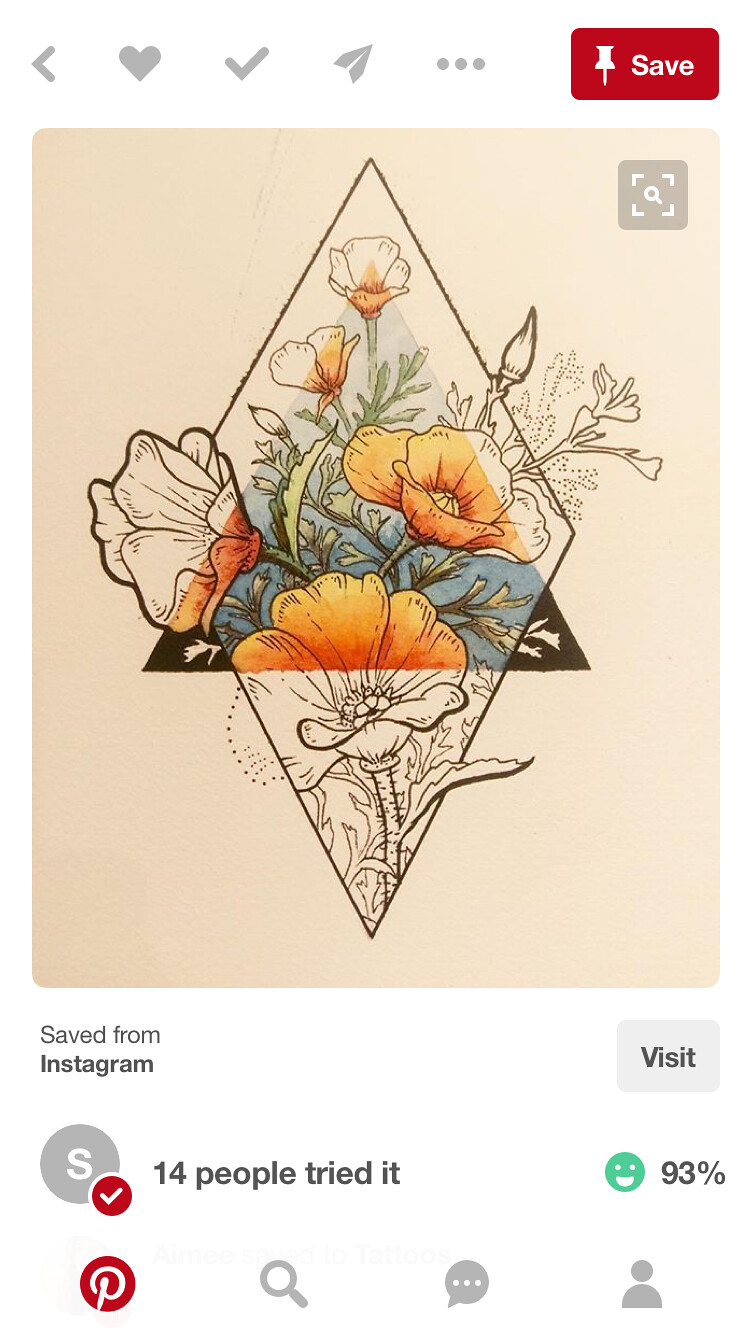In this image, we see a detailed screen capture of an Instagram post featuring an illustration of floral artwork, which appears to be from Pinterest but has interface elements from both Instagram and Pinterest. The background of the artwork is a gradient peach or light pink that is darker on the left and lighter on the right. Central to the image is a black outlined diamond shape with a partially obscured black triangle inside it. The middle of the diamond showcases vividly colored flowers - mainly orange blooms with blue and yellow centers, complemented by green leaves and stems. These flowers are fully colored within the diamond’s center, while floral outlines extend beyond the diamond in just black ink.

Above the illustration are Instagram's typical interactions icons: a gray arrow pointing left, a heart, a checkmark, a paper airplane-shaped share button, three dots, and a prominent red 'Save' button featuring a white pushpin. Below the artwork, there is a gray and white 'S' button accompanied by the text "14 people have tried it," marked with a red circular checkmark. Another element is the Pinterest logo, a white and red cursive 'P,' followed by a gray search magnifying glass, a gray and white chat bubble with three dots inside, and a gray and white outline of a person. Directly above these icons is a green circular smiley face with "93%" written next to it. Further up, there are the words "Save from Instagram" on the left and a "Visit" button on the right.